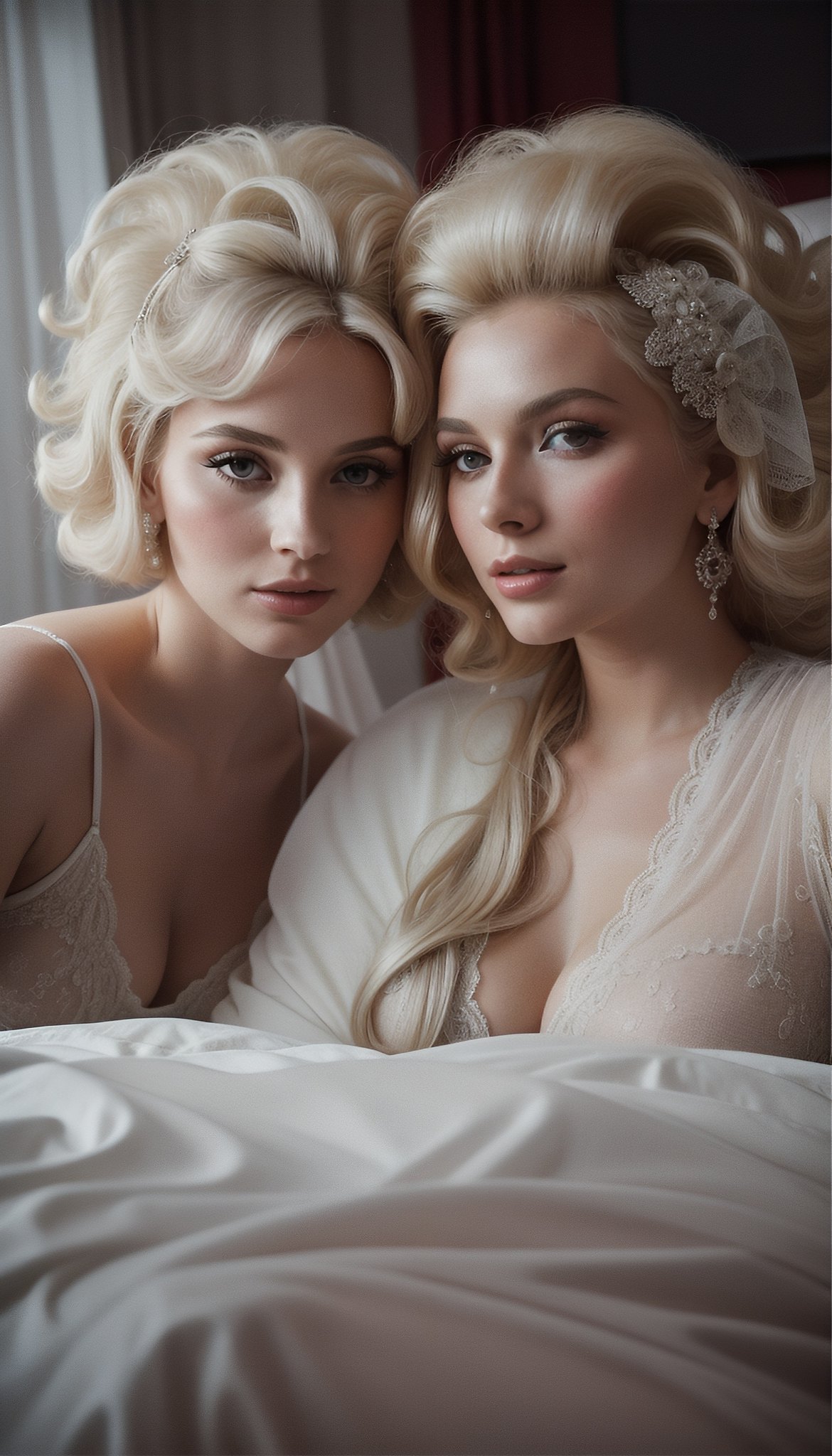This is a narrow, vertically aligned rectangular photo featuring two women with distinctive blonde hairstyles. The woman on the left has short, curly, very blonde hair, while the woman on the right sports long, blonde hair that is styled with a comb-over at the top and cascades over her right shoulder past her chest. Both women are gazing directly at the camera, showcasing their makeup and similar facial features.

The woman on the left is wearing what appears to be a white, lacy spaghetti-strap top with a low-cut neckline, possibly lingerie. The woman on the right is adorned in a white, lingerie-style nightgown with lace trim at the top and a silvery hairpiece. Their heads are touching, with the left side of the woman on the left’s head pressed against the right side of the woman on the right’s head, suggesting an intimate closeness.

It’s unclear if the woman on the right is seated on a chair or bed while the woman on the left leans in against her. The background features white curtains, contributing to an indoor setting that may suggest a professional photo shoot or a personal portrait session.